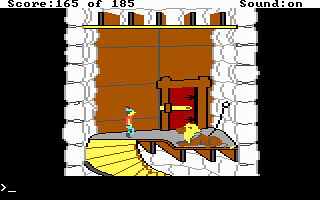The image depicts a pixel art style screenshot from a game. At the top of a flight of yellow stairs on a gray platform, a character engages in conversation with a creature that is resting on all fours. This creature has a brown body, a yellow head with a brown mouth, and something possibly atop its head. It appears to be chained to the wall.

Flanking the character and the creature are white stone walls, while in the background, there is a brown wall featuring a red door. The door is framed with thick brown wood and has a yellow latch, suggesting it is locked. The door also has black brackets for additional detailing.

Surrounding the central gameplay area is a black border, indicating the limits of the game's display. At the top of the image, a white banner stretches across the screen, showing black text that reads "Score: 165 of 185," followed by a large space, and then "Sound: On."